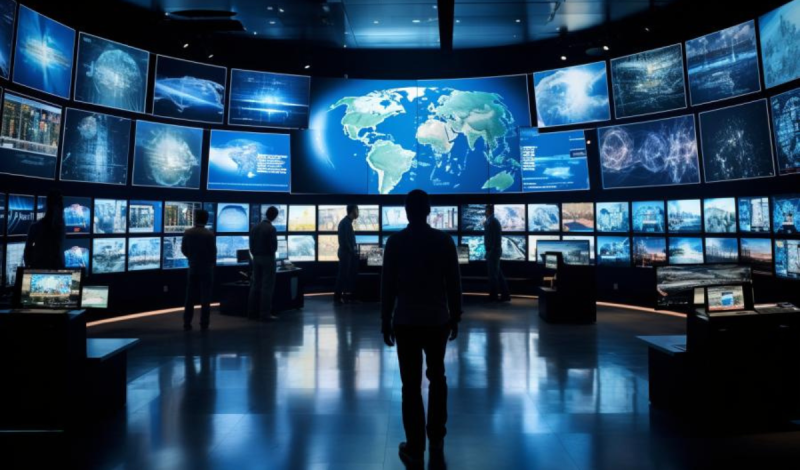The image depicts a dramatic, futuristic newsroom with a curved wall filled with various screens displaying an array of sci-fi visuals. Dominating the center is a large screen featuring a map of the world, flanked by smaller screens showing intricate digital images and buildings. Below these are even tinier screens, creating a layered visual effect. In the foreground, a person appears as a black silhouette due to intense backlighting, standing amidst reflective, smooth tiles that mirror the scene above. Surrounding this figure are several others, also dark silhouettes, intently facing the screens. Some people are seen with giant laptops, suggesting a high-tech environment. The entire setting exudes a clean, polished look, akin to a film set or an advertisement rather than a real-life location.